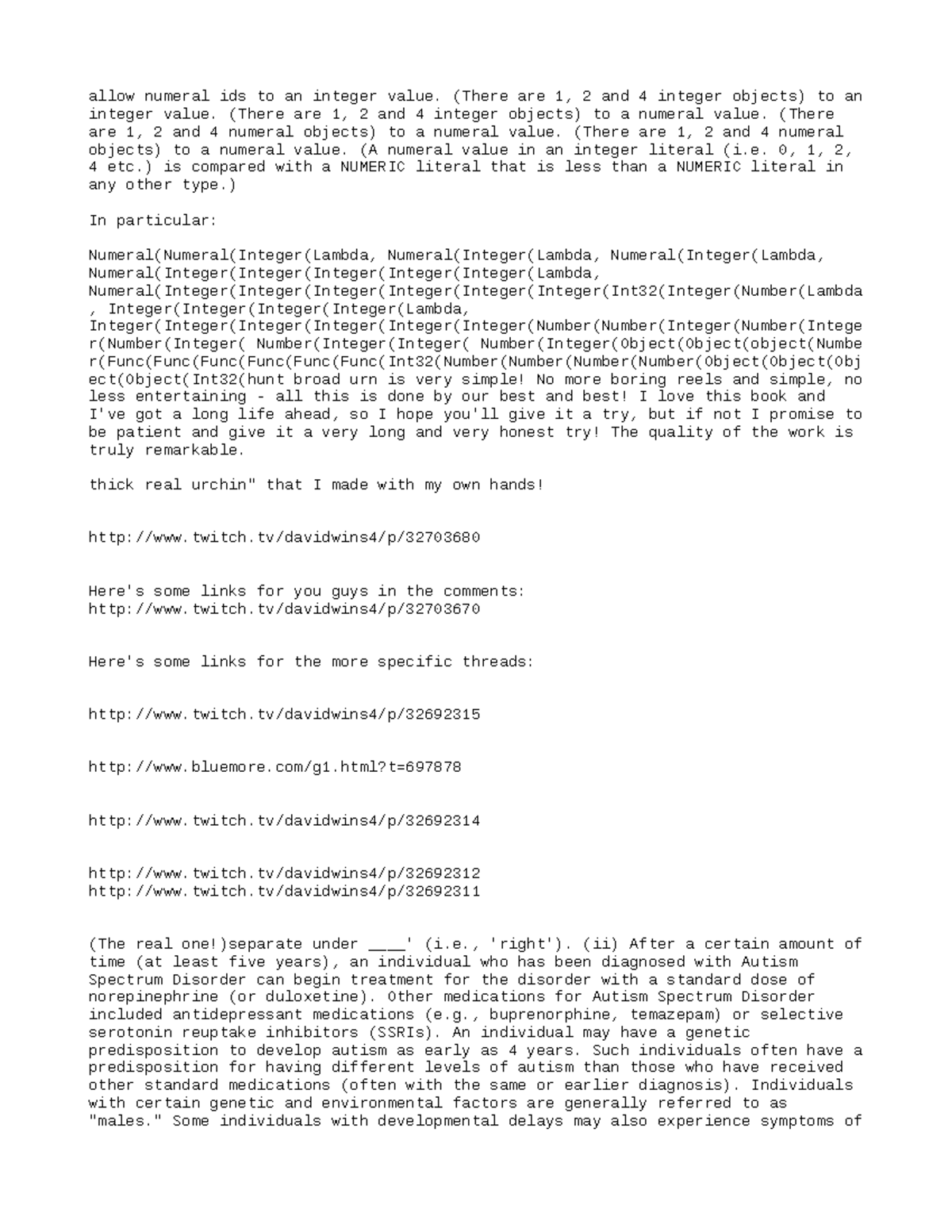This is a detailed screenshot showing several segments of HTML code, written in Courier-style font in black against a white background. The first segment of the code specifies, "Allow numeral IDs to an integer value (there are 1, 2, and 4 integer objects) to an integer value (there are 1, 2, and 4 integer objects)." The code then continues with the sentence "There are 1, 2, and 4 numeral objects to a numeral value," which is repeated for two additional lines.

The next part of the code begins with "In particular:" followed by a long paragraph. This section contains several lines of repetitive pseudocode-like structures, such as "numeral (numeral (integer (lambda, numeral) integer (lambda, numeral) integer (lambda, numeral)..." continuing for several lines.

Following this complex code section is a line of text that reads, "Broad urn is very simple! No more boring reels and simple, no less entertaining—all this is done by our best and best! I love this book and I've got a long life ahead, so I hope you'll give it a try. But if not, I promise to be patient and give it a very long and very honest try! The quality of the work is truly remarkable."

Further down, there are some links in the text, including URLs to twitch.tv and additional text that might describe aspects related to autism. The overall context is somewhat nonsensical and seems to be a mixture of placeholder code and unrelated text, all formatted in HTML.